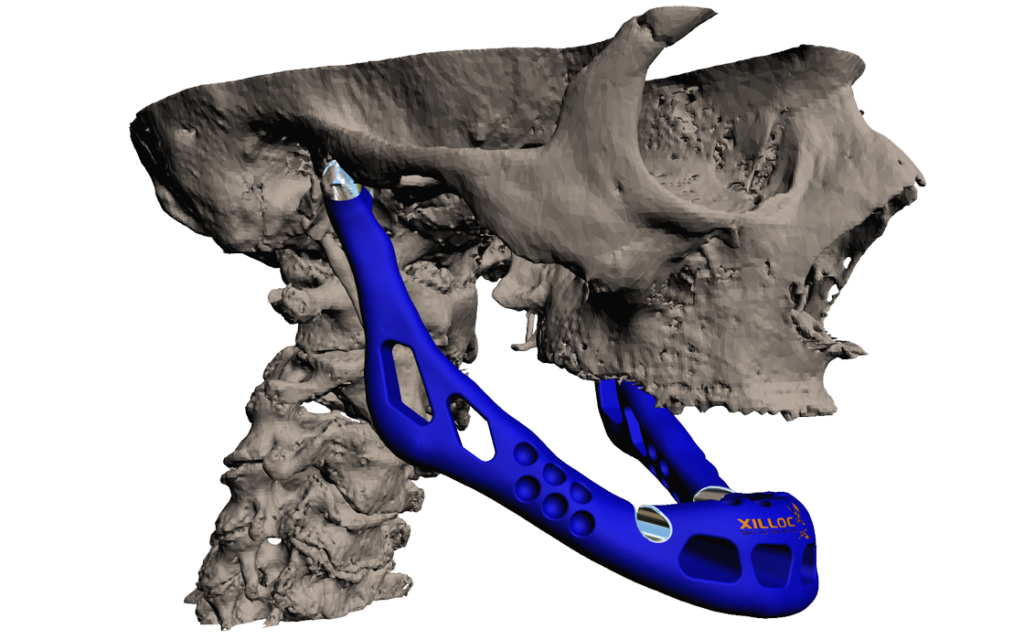This image features the bottom portion of a human skeleton's skull, specifically showcasing a missing jaw. The gray skull is partly cut away, revealing the eye sockets, nasal cavity, and the upper mouth area. Attached to the skull is a bright blue, 3D-printed titanium jaw, labeled with the word "XILLOC." This artificial jaw, likely intended for dental or medical implantation, connects to the skull near the base of the ears and extends downwards. The bright blue jaw contrasts sharply with the skeleton’s natural bone color. The jaw includes multiple small holes, has a silver attachment point, and bears the label "XILLOC" in dark yellow letters on the front. The skeleton's neck vertebrae are also visible, descending from the base of the skull.